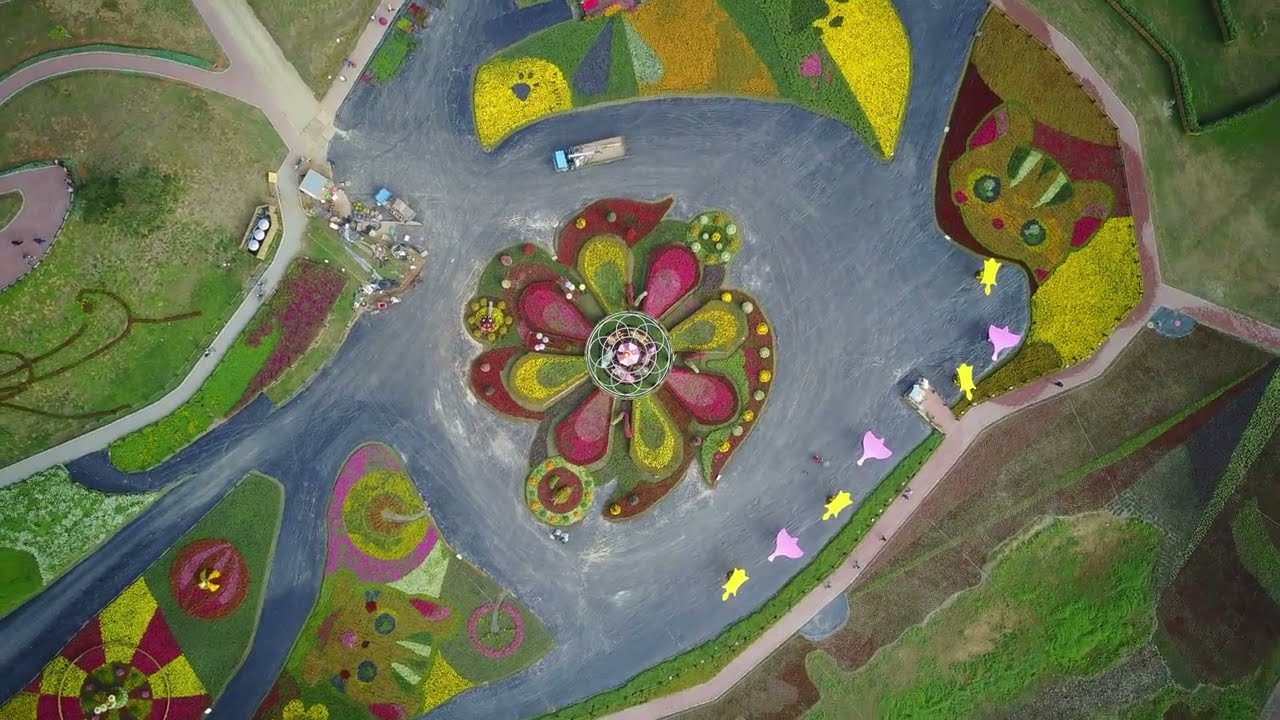This vibrant and abstract artwork features a central decorative flower with pink, green, and yellow petals and a small green circle in the middle, set against a blue background. Surrounding the flower are various whimsical elements, including colorful drops of yellow, orange, and brown. Towards the top right of the painting is a playful representation of a yellow and green bird-like figure, while the top left features another object adorned with cat paws. The entire composition gives the impression of a landscape seen from above, with gray pathways winding through a stream-like area. Scattered throughout are several islands, each with its own distinct features such as cat faces in the upper right and lower middle, as well as green cat paw prints in the upper left. The artwork is framed by two solid black rectangular areas on the sides, enhancing the abstract and playful nature of the piece.